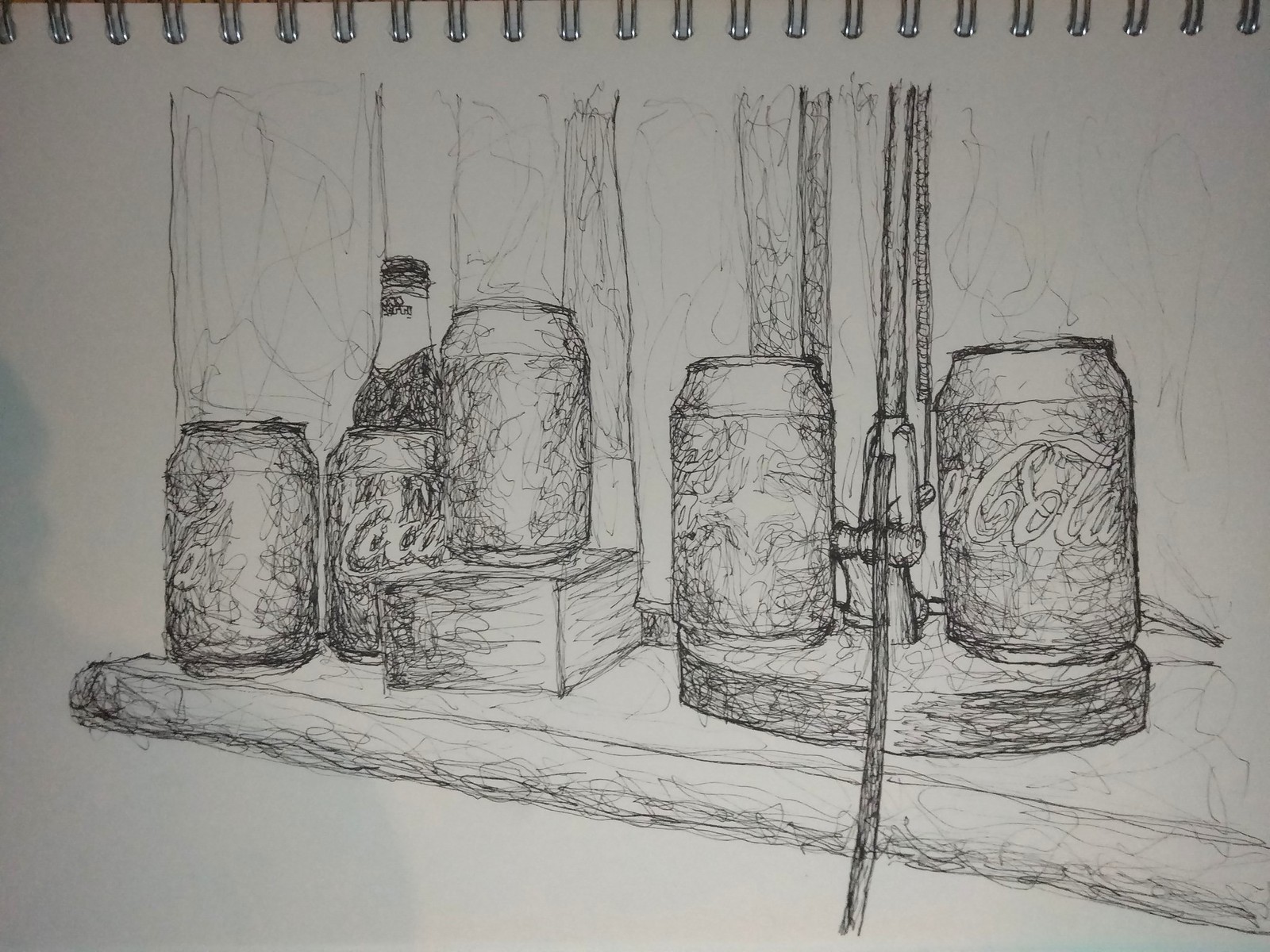The image depicts a white notebook with multiple silver rings binding it at the top. In the center of the drawing, there is a large platform holding several cans and drinks. On the right side, a circular platform is noticeable, and above it, there is an object with cables extending from its side. To the left of the main platform is a single can, and to its right is a can of Coca-Cola. In the background, numerous lines create an intricate backdrop. Further to the left of the Coca-Cola can, another can is depicted, followed by a bottle of Coca-Cola, and then yet another can. One of these cans is positioned atop what seems to be a block. The entire illustration is drawn with pen and shaded using an array of curvy lines, giving it a dynamic and textured appearance.